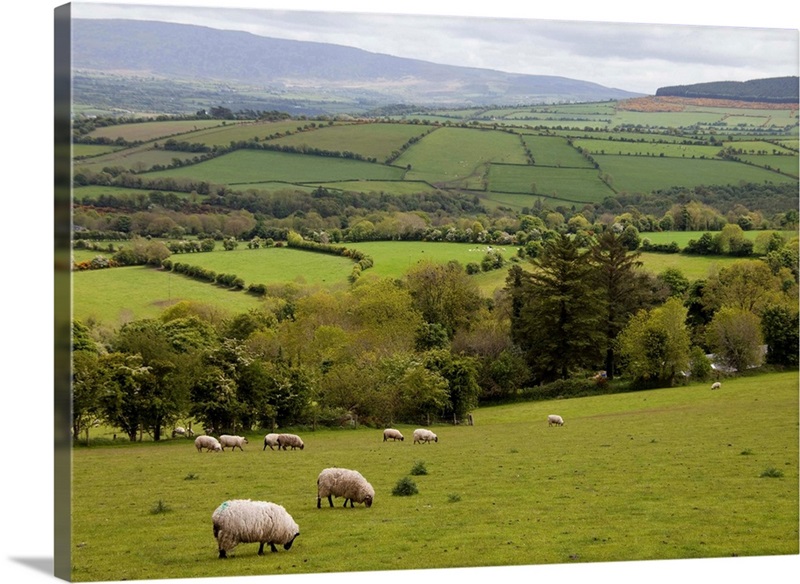The image captures a picturesque and meticulously groomed landscape, likely situated in Britain or Europe, with a strong possibility of being Wales. It showcases a vast, green expanse composed of fields separated by tree lines, extending into the distance where low mountains and hills form a scenic backdrop. The fields, varying in shapes and sizes, exhibit different shades of green and appear to be low grass crops or grazing areas. 

In the foreground, a number of woolly sheep, adorned with their white coats and black legs, can be seen grazing, some facing right, adding a lively touch to the serene scene. The neat, manicured look of the landscape is accentuated by the orderly tree lines and diverse tufts of trees, enhancing the overall beauty and tranquility of the view. In the distance, faint outlines of buildings emerge, contributing to the idyllic rural charm. The cloudy banks on the horizon add a soft contrast to the green of the fields and trees. The image is a testament to pastoral beauty, with flocks of sheep dotting the lush, rolling fields that stretch out towards the hills and valleys beyond.